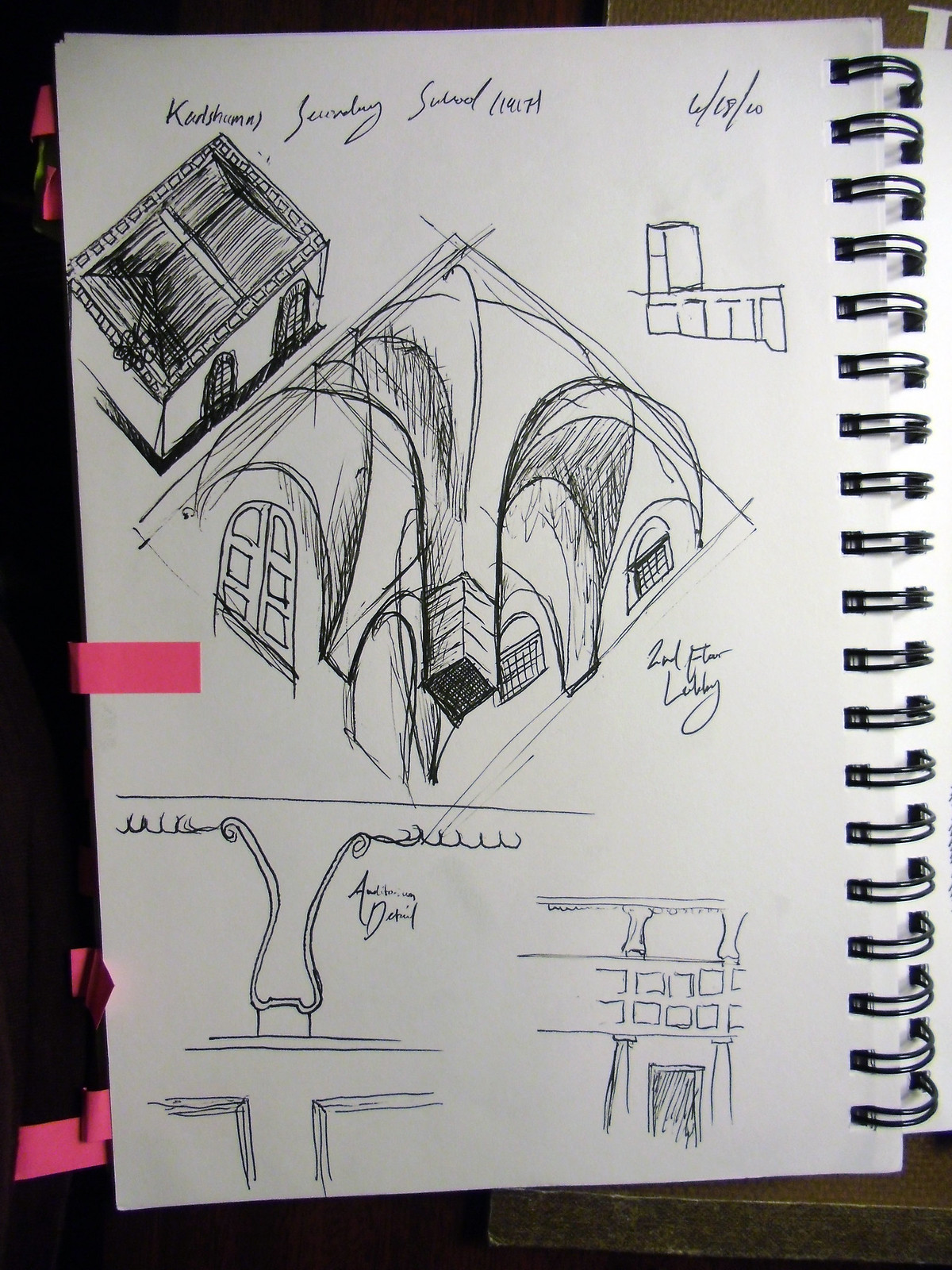The image features a detailed architectural sketch on unlined sketch paper within a black spiral-bound sketchbook, oriented so that the binding is along the right side. The notebook itself rests on a dark brownish desk surface. Pink post-it notes are visible along the left edge of the sketchbook, with one particularly prominent note folded across the page.

The focal point of the drawing is the "second floor lobby," prominently featuring a diamond-shaped (square turned on its side) sketch containing abstract images of arches and windows. A fine, loopy cursive script appears at the top of the page, somewhat slanted, with a partially legible date reading 6-18-10.

In the upper left corner of the page, there is a bird's eye view of a building's roof, showing two large wall-length windows. The structure is further detailed with fine black lines and smaller rectangles on the edges, suggesting bricks. 

The lower portion of the page seems to capture the living space or an intersection with designs perhaps intended for artwork installations or street designs, featuring a base with a V-shaped structure that resembles a fountain emanating steam, indicating an entry labeled as "auditorium detail." 

The intricate sketches in dark ink include detailed images of paneling, windows, possibly a fireplace, and elaborate architectural elements like a pillar morphing into an archway that connects to the ceiling – all indicative of a meticulous architectural schematic laid out by what appears to be an architecture student.